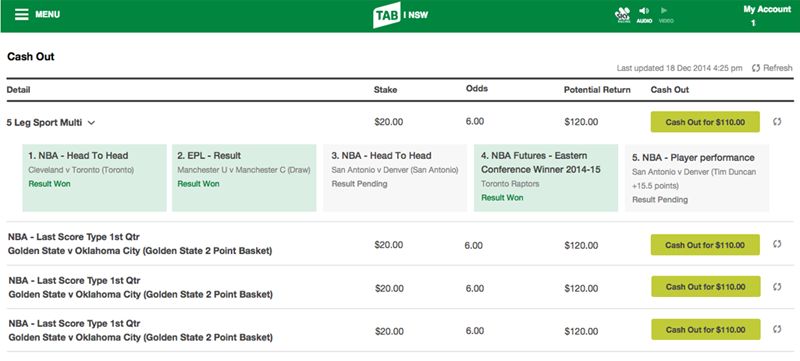Here's a detailed and cleaned-up caption for the image:

---

This image features a detailed view of a sports betting menu. At the top, a green bar spans horizontally with the main navigation options displayed, including a contacts menu on the left side. The central menu is organized into sections such as "Tab I-N-S-W," "Audio Video," "My Account," and it shows the user’s current bets and winnings. 

Key bet details are shown with sections labeled "Legsport Cashout Options," "Details," "Your Stake," "Potential Return," and "Cashout Option."

The listed bets include:
1. A multi-leg sports bet featuring:
   - NBA head-to-head: Cleveland vs. Toronto (Result: Win)
   - EPL result: Manchester vs. Manchester City (Result: Draw)
   - NBA head-to-head: San Andres vs. Denver (Result: Pending)
   - NBA Futures Eastern Conference winner: Toronto Raptors (Result: Win)
   - NBA player performance: Tim Duncan, 15.15 points (Result: Pending), with a cashout option of $110.

2. Another series of bets for the NBA first quarter:
   - Golden State vs. Oklahoma City, $20 stake, 6.0 odds with a $120 potential return and a cashout option of $110.
   - A repeated bet for Golden State vs. Oklahoma City, $20 stake, 6.0 odds with a potential return of $200.
   - Yet another bet for the same event, $20 stake, 6.0 odds with a potential return of $120 and a cashout option of $410.

Overall, this is a comprehensive view of a sports betting website, showing the various bets placed, their results, and potential cashout options.